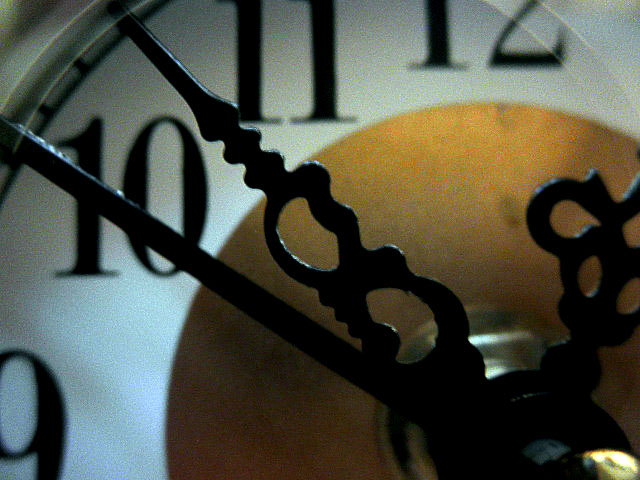This close-up image captures the intricate details of a clock, likely a vintage grandfather clock given the spacious arrangement of the hands and numerals. The image prominently displays the numbers 9, 10, 11, and 12 in a casual, yet elegant font set against a pristine white background. Central to the clock face, there's a gold or bronze circle, marking the attachment point of the beautifully crafted clock hands. The combination of intricate craftsmanship and tasteful design elements suggests a blend of functionality and aesthetic appeal, encapsulating the timeless charm of a classic timepiece.